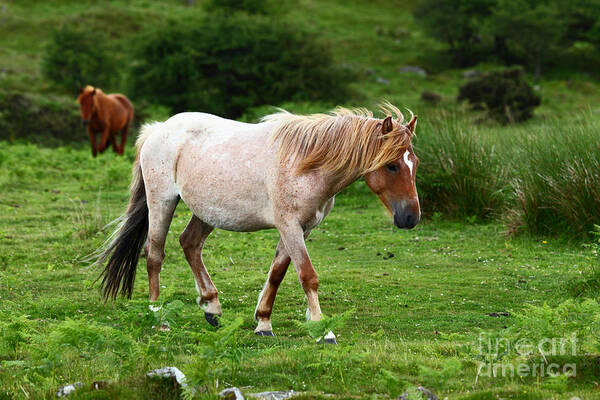This outdoor daytime photograph, taken on an overcast day with no visible sun or shadows, showcases two horses in a lush, green landscape of fields, bushes, and trees. In the foreground, a brown and white horse walks from the left to the right. This horse features a dark brown face with a distinctive white patch between its eyes, a mostly speckled white body with brown spots, a brown mane, and a darker tail. In the background, a solid dark brown horse approaches from a slight incline, partially obscured and out of focus. The grassy area varies from short grass in the immediate foreground to tufts and clumps of taller grass, small trees, and shrubs in the distance. The photograph is marked with the Fine Art America watermark in the bottom right corner.